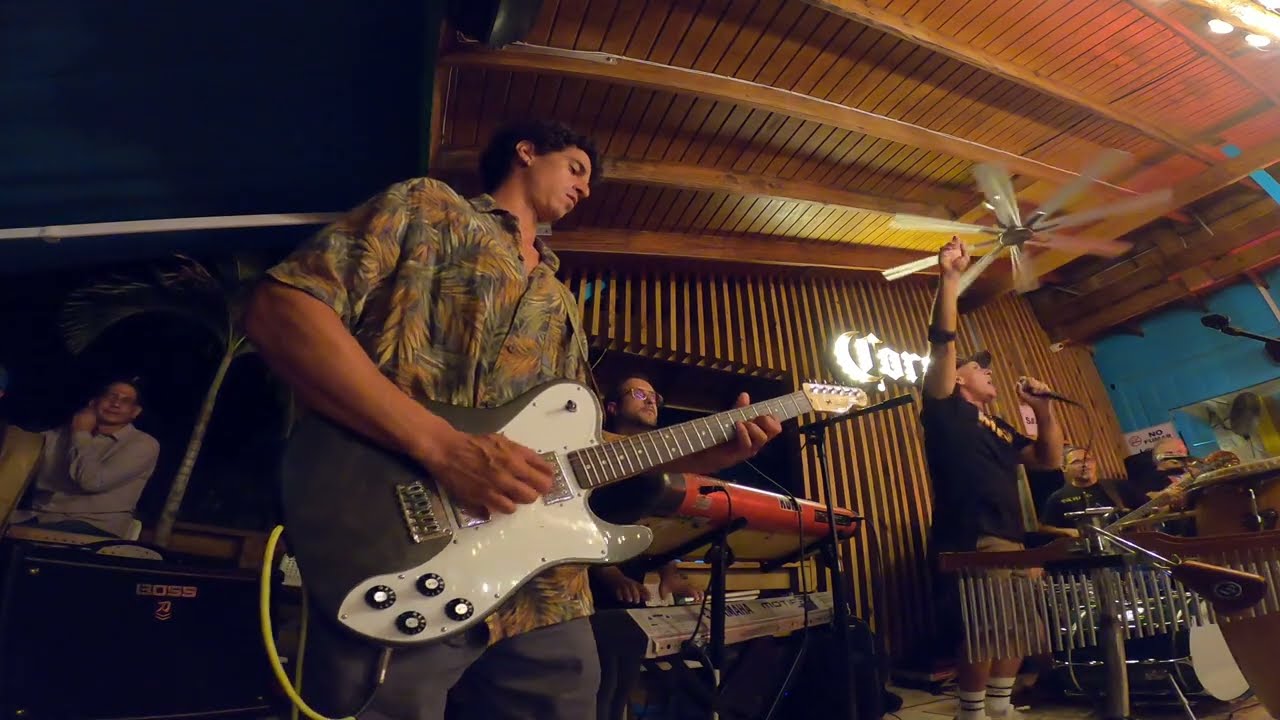In this image, we see a band performing, likely indoors at a bar or restaurant with a live music setup. Central to the scene is a guitar player clad in a tropical shirt and gray shorts, playing a gray Fender Telecaster Deluxe with a white pickguard and chrome square humbucker pickups. To his right, a keyboard player operates a red keyboard with a gray one below it. Further right, a vocalist with his arm raised holds a microphone, and in front of him, a chime-like instrument or xylophone can be seen. In the right-hand corner, a drummer is visible, rounding out the band ensemble. The setting suggests an indoor venue, featuring a wooden pavilion-like ceiling with a fan, and the backdrop includes a Corona beer sign and various lights, enhancing the musical atmosphere.